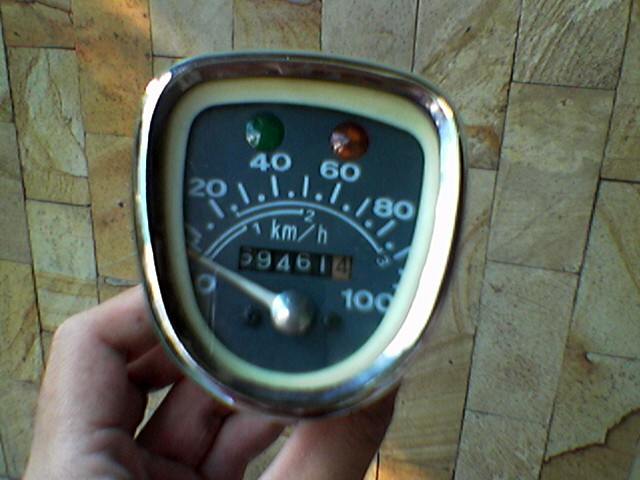This photograph features a vibrant, multi-colored tiled background, composed of a mix of gray, brown, and brown tiles adorned with gray decorations. From the bottom of the image, a Caucasian hand enters the frame, gripping what appears to be a speed-measuring device or thermometer. The instrument's sleek design includes a silver body, encased by a white border and further accented with gray. At the bottom of the device, a silver needle points towards zero, aligning with a scale marked with numbers in increments of twenty: 0, 20, 40, 60, and 80.

Just above the scale, the device boasts a single green light and a red light. Additionally, a section with a black background displays white numerical digits arranged in pairs: 6, 9, 4, 6, 1, 4. The combination of the detailed tiled backdrop and the intricate features of the handheld device make for a visually engaging photograph.